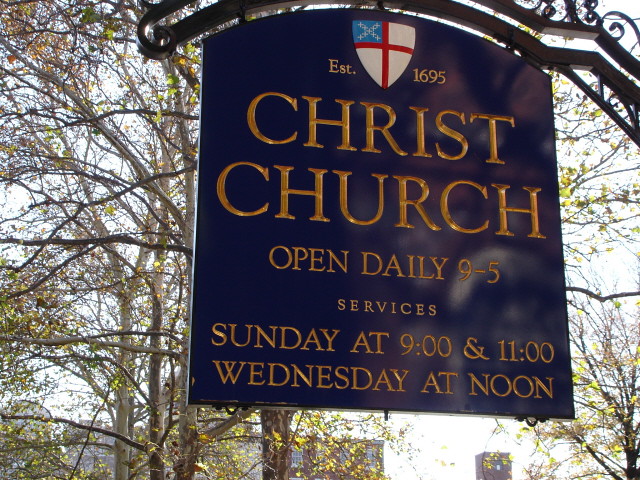This photograph captures an ornate, navy blue sign hanging from an intricate black iron post. The sign is square with an arched top, adorned with a prominent shield at its center. The shield features a white background with a red cross, and the upper left quadrant is blue with a white X. Flanking the shield, the text "Established 1695" is written in gold lettering. Below the shield, "Christ Church" is prominently displayed in large gold capital letters, followed by the schedule "Open Daily 9-5," "Services," "Sunday at 9 and 11 o'clock," and "Wednesday at noon." The background reveals a picturesque scene with trees and buildings.